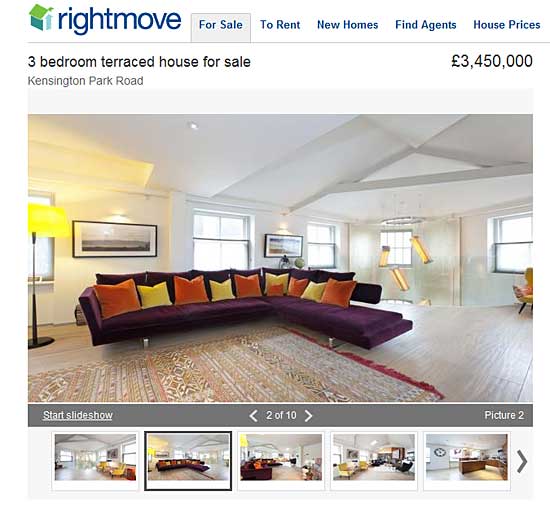The image is a promotional advertisement for the website Rightmove, showcasing a property for sale and highlighting options for renting new homes, finding agents, and viewing house prices. The property featured is a charming three-bedroom terraced house located on Kensington Park Road, listed at £3,450,000. 

The room displayed in the photograph exudes a spacious and airy atmosphere, accentuated by its tall ceilings and large open windows that allow natural daylight to flood in. The decor is sophisticated with white walls and elegant light brown hardwood floors. A beautiful purple couch adorned with a mix of orange, yellow, and sequin pillows stands as the centerpiece, enhancing the room's inviting and vibrant ambiance. 

Adding to the room's charm, a sizable rug complements the light tan flooring, while a striking lamp with a big yellow shade and long, rectangular pictures on the walls enhance the overall aesthetic. The image is part of a slideshow, currently displaying picture two out of ten. The slideshow also includes the option to view five different rooms within the house, with this particular room being highlighted.

In the bottom left-hand corner of the screen, the Rightmove logo is visible, featuring an icon of a house with a green roof, blue siding, and a light blue door, symbolizing the website’s brand and its services.